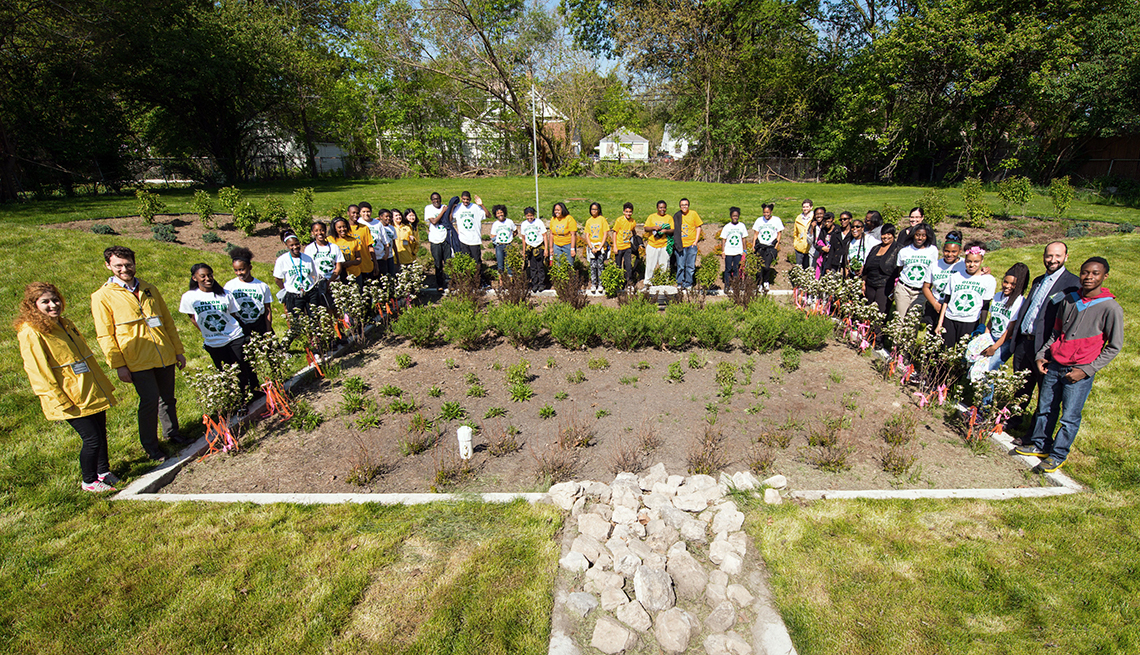This is a color photograph taken outdoors on a sunny day, capturing a vibrant community scene centered around a meticulously tended garden plot. The garden itself is a square, or possibly rectangular, section of land bordered with white stones and partially filled with large white rocks that form a path extending from its base. Within this plot, rows of green vegetation and flowers are intentionally planted, showcasing an array of flowers along two sides and possibly vegetables in the main sections. 

Surrounding this garden on three sides is a diverse group of volunteers and students, suggesting a community or school-organized event. The majority of the students are wearing white t-shirts adorned with a green recycling logo, indicative of environmental or recycling efforts. A noticeable number of participants also don matching yellow t-shirts, while some adults and other attendees wear regular street clothes. The backdrop features trees and residential structures, including homes and garages, under a clear sunny sky, enhancing the vibrant and lively atmosphere of this communal activity.